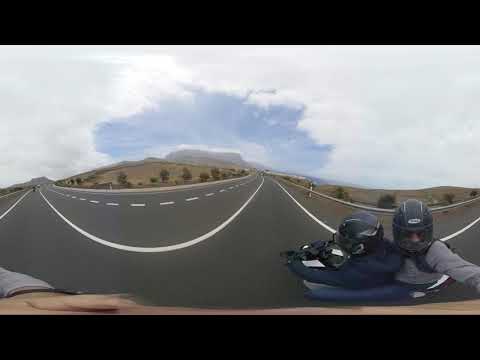The image captures two individuals riding a sleek black motorcycle down an open, well-paved road that stretches into the horizon, with white lines neatly marking the lanes. Both riders are clad in black helmets for safety. The motorcyclist driving wears a blue sweatshirt and firmly grips the handlebars, while the passenger, dressed in a gray sweatshirt and blue jeans, holds up a camera or GoPro, revealing a black watch on their wrist. The expansive landscape around them features a predominantly brown, arid terrain with scattered dark bushes that suggest a dry and possibly hot environment akin to a desert. Far in the background, a distant mountain or plateau rises subtly under a light blue sky adorned with a few white clouds. The image is somewhat distorted, giving it a panoramic appearance with exaggerated curves, adding to the sense of a remote, endless road in the middle of nowhere.